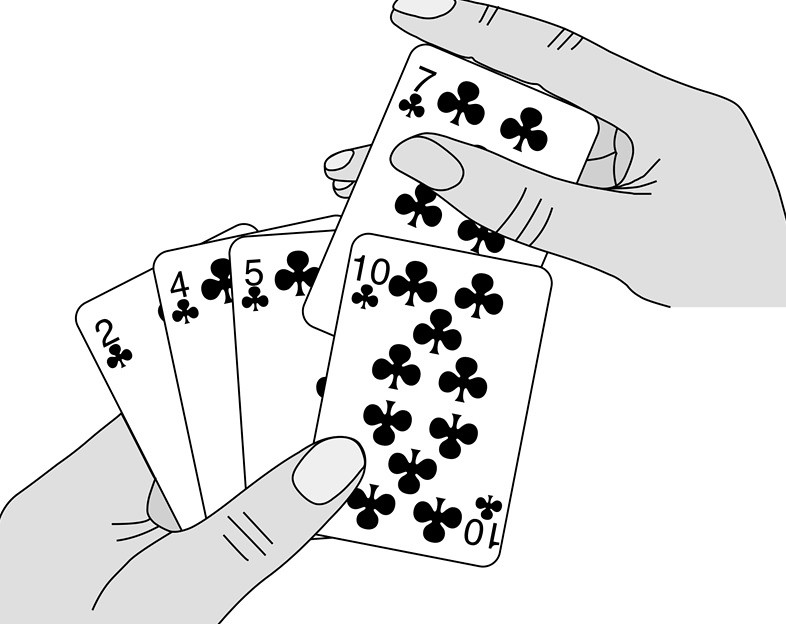This black and white illustration, which resembles a photograph but possesses the intricate detail of a line drawing, features a minimalist white background. The primary focus is on a pair of hands holding playing cards. The left hand, located in the lower left corner, reveals a thumb only, suggesting an intimate, close-up angle. Positioned in the upper right, the right hand displays a thumb, a visible finger, and the edges of two other fingers, giving a sense of partial concealment.

Intriguingly, the bottom portions of both hands fade out as if they were abruptly cut off, adding an abstract element to the composition. The hands themselves are defined by dark, precise lines, which create a striking contrast against the white backdrop. However, the outlines dissolve at the bottom, blending seamlessly with the background.

Between the hands are five playing cards, arranged in a fan-like spread. The left hand holds a two of clubs, a four of clubs, a five of clubs, and a ten of clubs in a splayed display, revealing the full face of the ten of clubs and the left edges of the remaining cards. The right hand is in the motion of drawing a card from the spread, specifically a seven of clubs positioned between the five of clubs and the ten of clubs. The seven of clubs, partially extracted, is still nestled between the fingers of the right hand, adding a dynamic touch to the otherwise steady presentation.